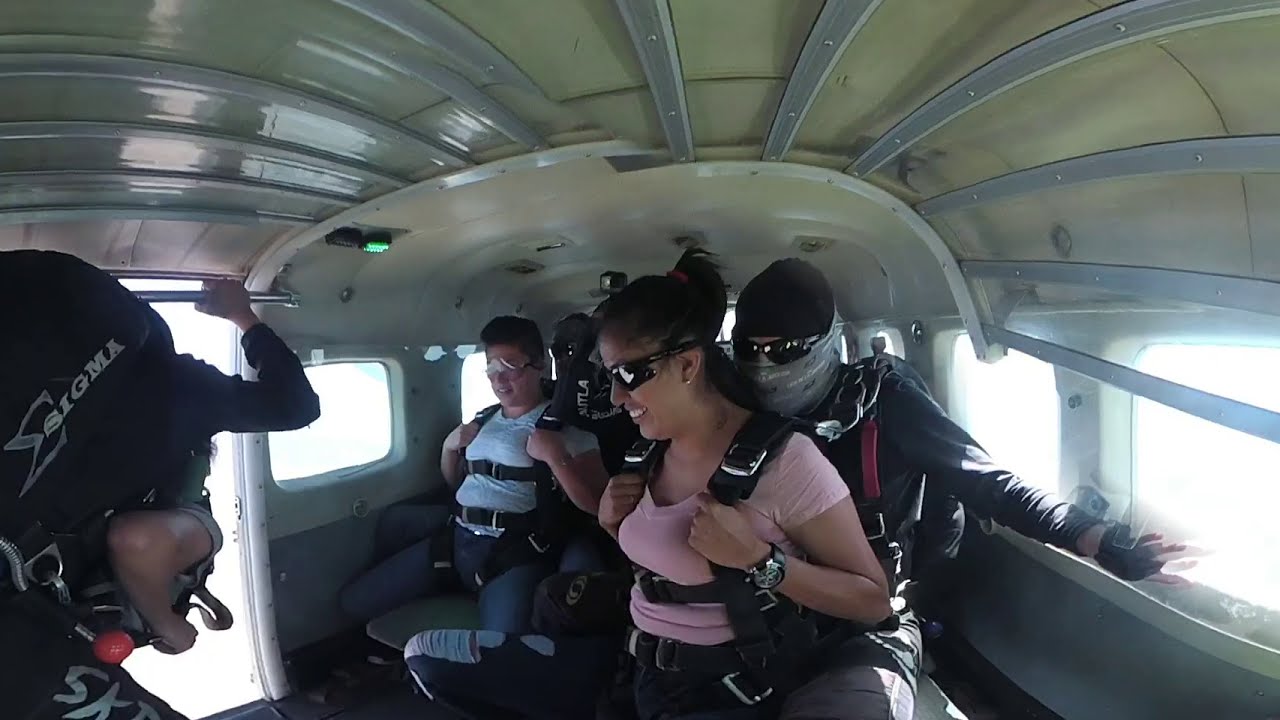In this detailed photograph, four individuals are seated inside a smaller aircraft, likely a chartered plane or helicopter, in preparation for a skydiving adventure. All occupants are securely buckled in and wearing skydiving gear, including safety glasses. The focal point is a woman in a pink shirt with her hair in a ponytail, looking both nervous and excited. She is harnessed to a male instructor behind her, who is distinguished by his bandana over his nose and mouth, black beanie, long-sleeve shirt, and safety gloves. To the left of the image, an instructor stands at the open doorway, ready for the imminent jump. The interior of the aircraft is white, accented by a green light at the top, and the other passengers include a man with a blue shirt by the window and another wearing a cap with the word 'Sigma' emblazoned on it. The scene, centered around the group, is set amidst a multitude of colors including brown, gray, green, black, white, red, pink, light blue, and purple, indicating the varied equipment and attire of those onboard. All are poised in anticipation of their skydiving experience, captured in a moment of readiness against the backdrop of a bright sky.